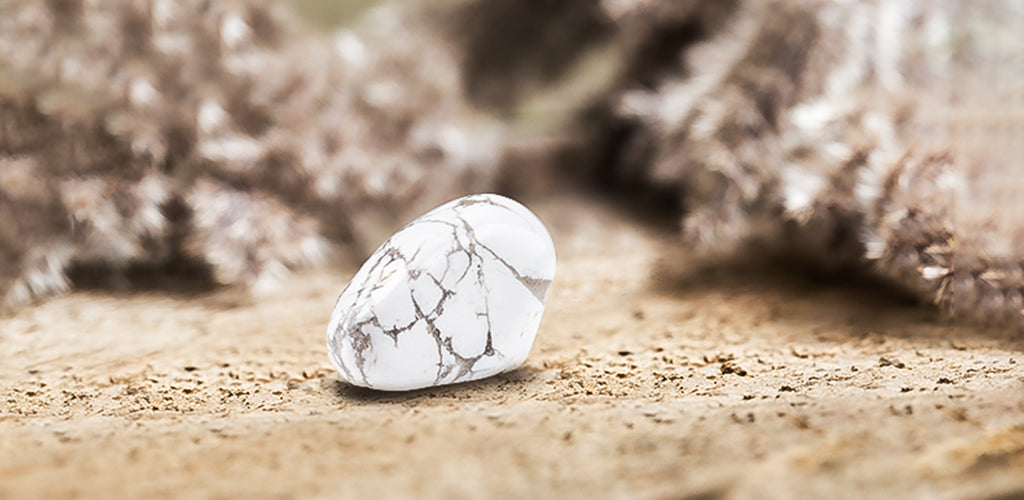This photograph captures a singular white rock, which resembles a tumbled stone or potentially a polished egg, sitting on a dirt ground. The rock has a distinct marble-like texture with light gray, possibly translucent, cracks and seams running throughout its structure. The image has a natural color palette dominated by browns, grays, and blacks, with no presence of greens or blues. In the blurred background, some brown rocks and potential silhouettes of trees or dead vegetation can be vaguely discerned. The ground is uniformly dirt, emphasizing the earthy tones of the image. The rock stands out prominently due to its bright white and gray coloration, and it leans slightly to the right with a small shadow beneath it. Its roundish shape is not perfect, adding to its natural and unique appearance.